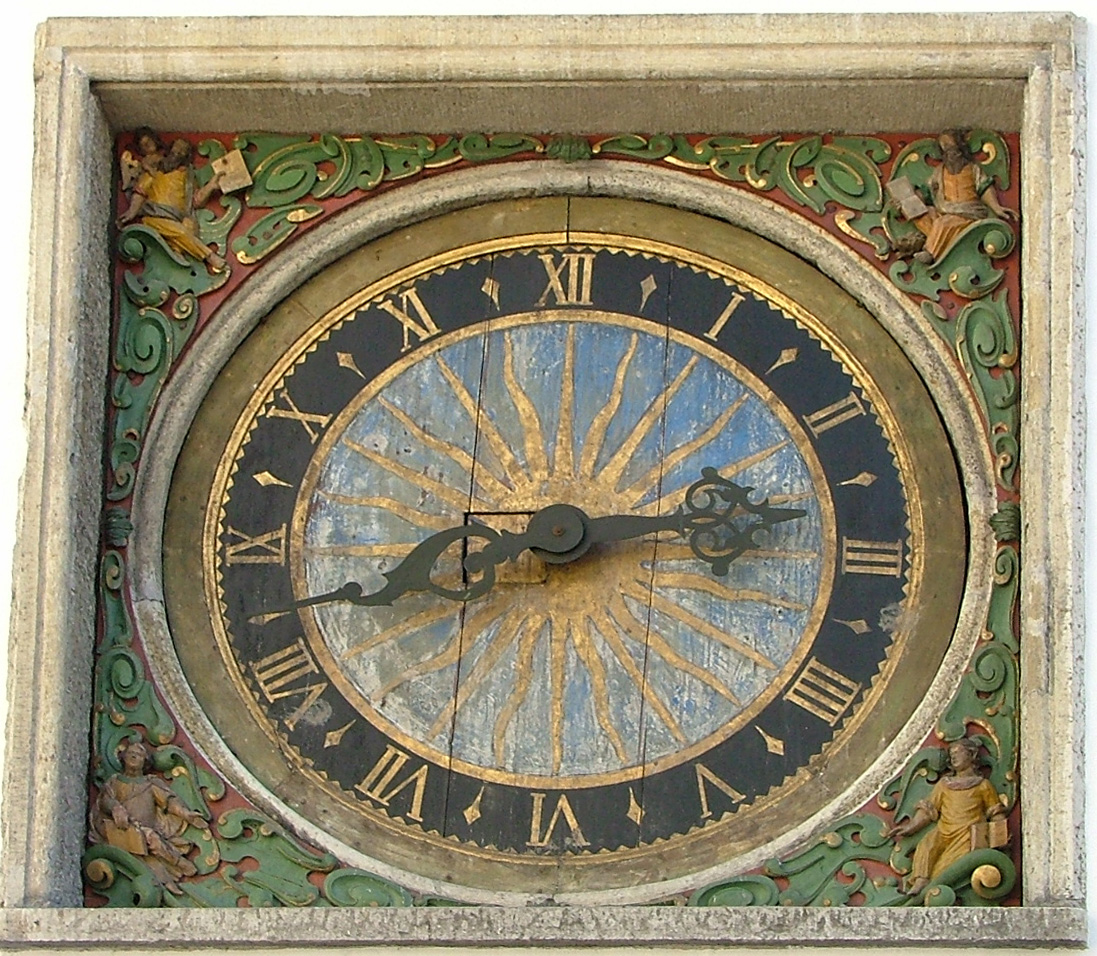The image features a beautifully detailed, very old analog clock encased within a square white stone or concrete frame, evoking an exterior architectural element. Within this frame, the clock is set into a circular, intricately carved wooden border that's vividly colored in green and red. This border is adorned with four figures, positioned at the upper left, upper right, lower left, and lower right corners, each resembling angelic or biblical beings dressed in flowing robes and possibly holding books. The clock face itself is encircled by a stone or concrete border, followed by a light tan stripe. The numerals on the clock are gold Roman numerals set against a black band. The center of the clock features a striking blue field adorned with a prominent gold sun, its radiant tentacles extending outward. The clock hands, made of wrought iron, include a larger and a smaller hand, both intricately designed. The combination of vivid colors, detailed carvings, and ornate figures creates a visually stunning and elegant appearance.